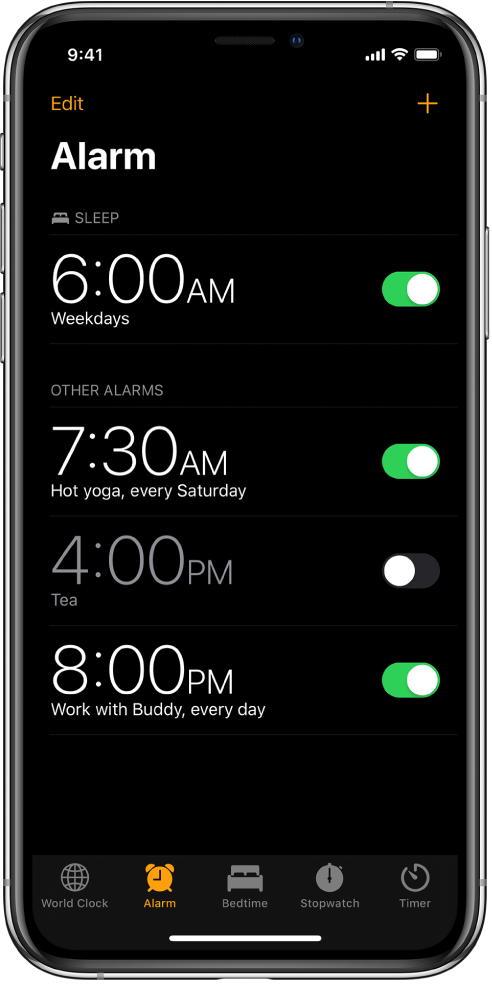Here's a detailed and cleaned-up caption for the image: 

"Screenshot of a phone's alarm page displaying four different alarms. The first alarm is labeled 'Sleep' and is set for 6:00 AM, with the toggle switch turned on to wake the user up during the daytime. The second alarm, named 'Hot Yoga,' is set for 7:30 AM and is activated for every Saturday. The third alarm, scheduled for 4:00 PM, is labeled 'Tea,' but its toggle switch is off. The fourth alarm is titled 'Work with Buddy,' set for 8:00 PM, with its toggle switch turned on for activation every day. Below these alarms, there are tabs labeled 'World Clock,' 'Alarm,' 'Bedtime,' 'Stopwatch,' and 'Timer.'"